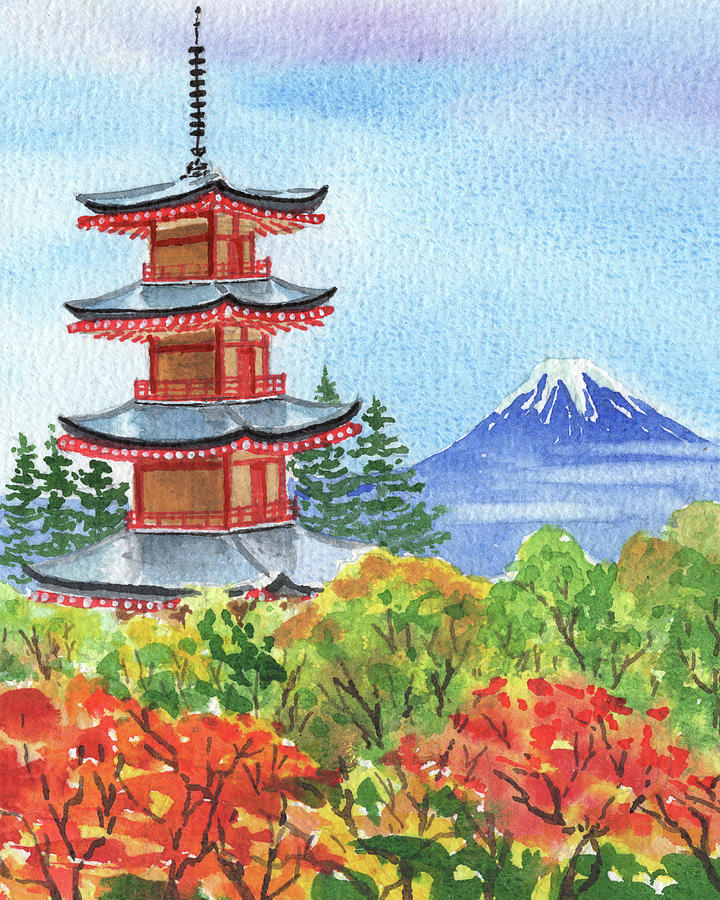This detailed watercolor painting showcases a traditional Japanese pagoda set against a stunning backdrop of Mount Fuji and a vibrant, seasonal landscape. Mount Fuji stands majestically on the left, its dark blue base capped with pristine white snow and partially veiled by delicate cloud cover. The sky above is beautifully rendered in smudged blue and white, typical of watercolor artistry. In the foreground, an array of foliage transitions from the green trees tinged with yellow, orange, and brown to striking orange fall leaves.

The pagoda, the painting's central focal point, is positioned on the right-hand side. It features a visible three out of its four stories, the lower parts obscured by the lush trees. The building itself has a striking brown structure with elegant red trim and red gates. The tiered roofs are black with red scalloped decorations, and a black antenna-like spire crowns the top. This traditional architectural marvel is complemented by surrounding green and orange plants that add to the depth and beauty of the scene.